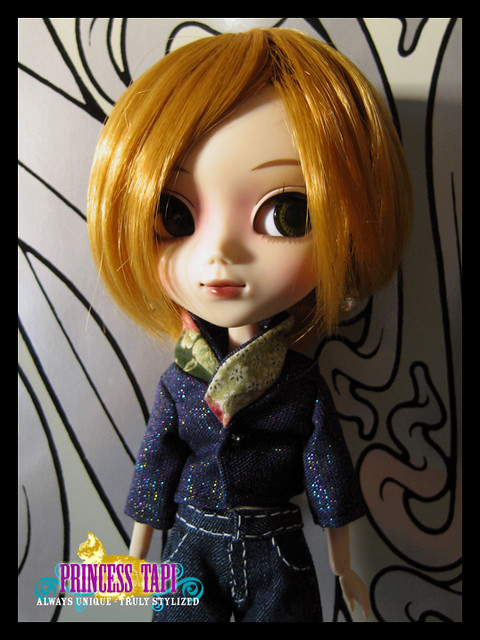The image features a children's doll centrally positioned against a wall adorned with an avant-garde abstract motif of gray and black swirls and shapes. The doll, resembling a young girl with pale skin and distinctly Asian facial features, has reddish-blonde hair that falls just above her shoulders and is complemented by dark pinkish-brown eyes. She is dressed in a sparkly blue top and blue jeans with white trim, although the image crops off at the upper legs, obscuring the lower part of her attire. Around her neck, she wears a green scarf or wrap. In the bottom left corner of the image, the text "Princess Tap" is prominently displayed in purple letters, accompanied by smaller, harder-to-read white text below it, possibly stating "Always unique, truly stylized." This text is overlaid on an image of a yellow cat.